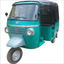The photograph depicts a quaint, old-fashioned, three-wheeled vehicle that resembles a cross between a golf cart and a jitney. This teal-colored vehicle features a front windshield with dual round side mirrors and a black windshield wiper. The front section boasts two headlights, a silver horizontal strip above them, and a dark gray plastic fender over the single front wheel. The back portion, covered with black leather canvas, has a wide bench seat that appears removable for an open-air experience. The back seat, protected by a screen to shield passengers from the wind, can be easily accessed via a step without the need for a door. The vehicle, which likely operates in urban settings offering short rides, is not road-legal due to its compact size and three-wheel configuration. The photograph primarily shows the left side of the vehicle, highlighting the left rear wheel and the intricate details of its design.